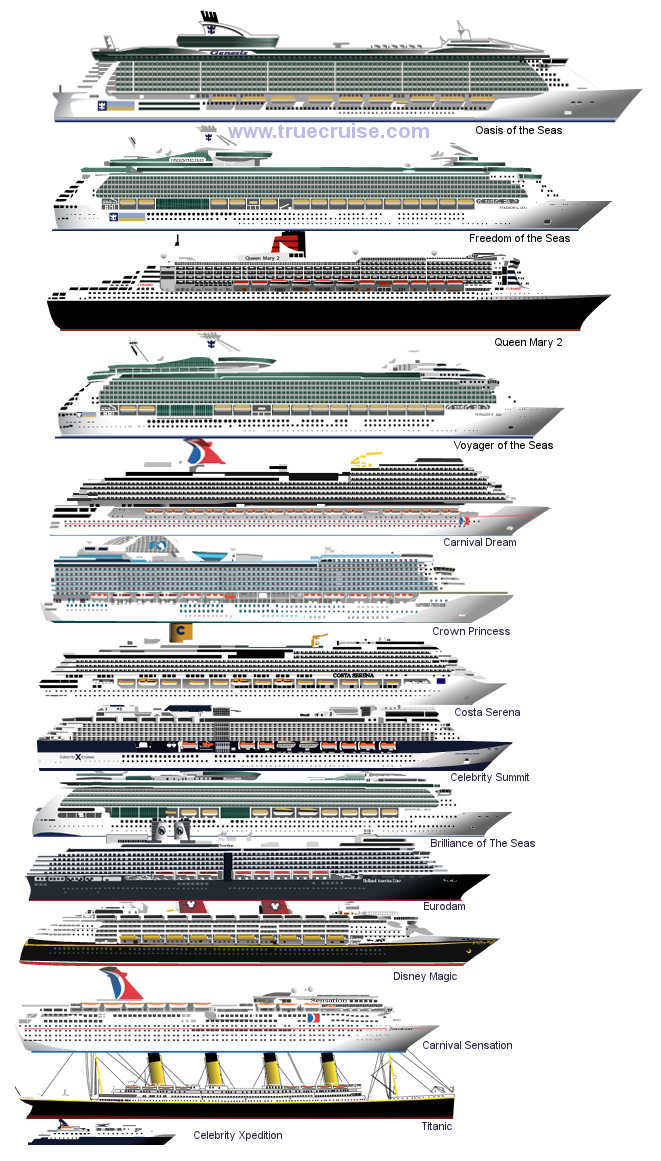The image is a detailed graphic representation of famous ocean line cruisers, arranged in a vertical column, showcasing the profiles of 13 or 14 ships. Each ship is depicted in a waterline sketch, showing only the superstructure above the water. The most modern and largest ships, such as Oasis of the Seas, Freedom of the Seas, and Queen Mary II, are positioned at the top, with progressively smaller and possibly older ships below them. Each ship’s name is listed in small text to the right of its profile. Notable ships in the list include Voyager of the Seas, Carnival Dream, Crown Princess, Costa Serena, Celebrity Summit, Brilliance of the Seas, Eurodam, Disney Magic, Carnival Sensation, and Celebrity Expedition. The image also includes a link at the top reading www.truecruise.com, indicating that this is an informational graphic aimed at conveying the sizes, makes, and models of these popular ocean liners to viewers.